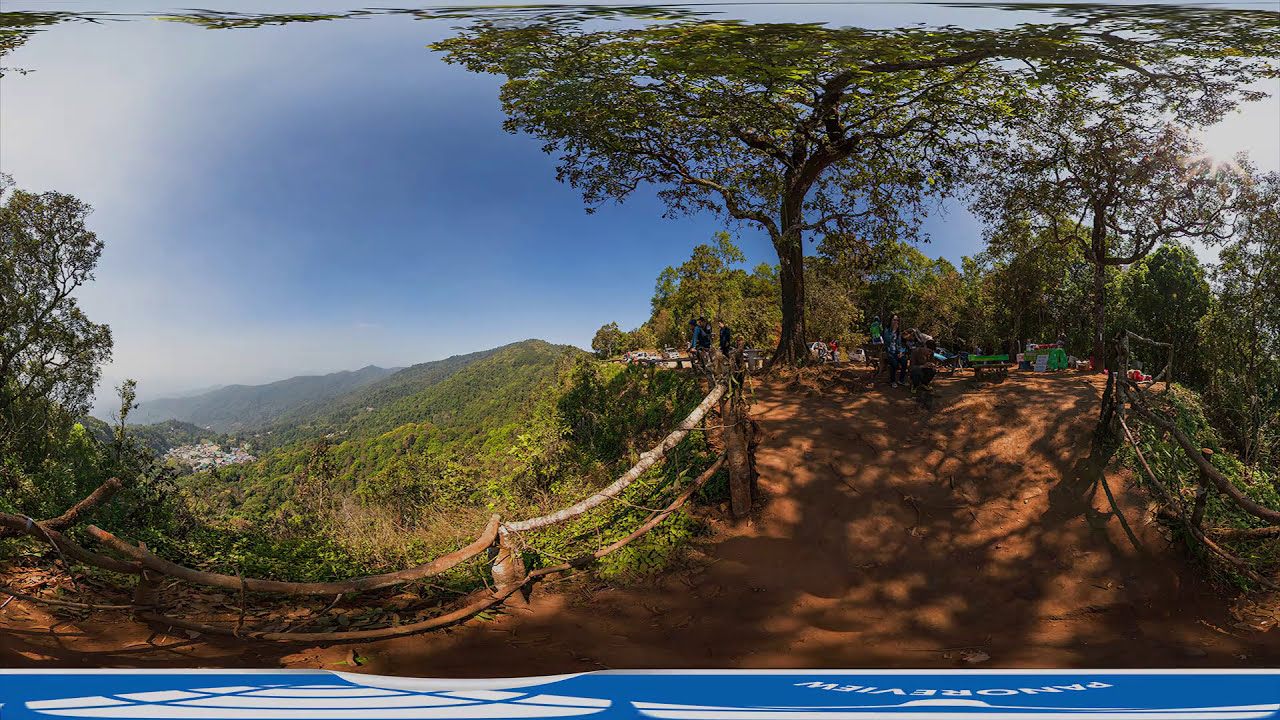In this panoramic view of a state park, a broad, rich brown dirt pathway stretches ahead, flanked by rustic wooden fences made of tree branches, logs, and posts on each side. The pathway, dappled with shadows from the overhanging trees, meanders slightly and ascends gently to the right. On the left side, the edge of the path precariously drops off over a cliff. The landscape is lush with trees, and in the distant background, low mountain ranges can be glimpsed under a blue sky. There's evident human activity with picnic tables, a green bench, lawn chairs, and a car park visible at the path's end. The image has a slight blur, possibly from a filter, and is horizontally rectangular, capturing this natural, serene environment with a sense of depth and texture.